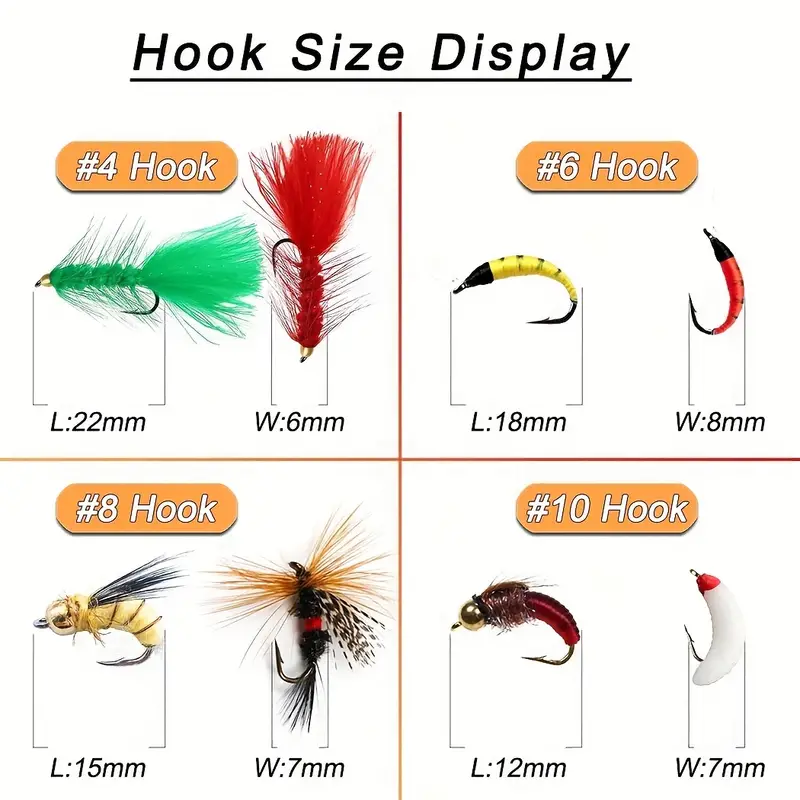The image is a detailed colored diagram titled "Hook Size Display" in underlined black letters at the top. It is divided into four quadrants with orange lines, showcasing different types and sizes of fishing hooks, each paired with vibrant fly designs. 

- In the top left quadrant, the number 4 hook, labeled with dimensions L 22 mm and W 6 mm, is adorned with insect-like flies featuring a green and a deep orange-red color.
- The top right quadrant displays the number 6 hook, sized L 18 mm and W 8 mm, which has flies resembling worms in yellow and red.
- The bottom left quadrant features the number 8 hook, measuring L 15 mm and W 7 mm, decorated with flies reminiscent of a bee.
- Lastly, the bottom right quadrant shows the number 10 hook, with dimensions L 12 mm and W 7 mm, styled with worm-like flies.

Each hook is displayed with detailed imagery, emphasizing their unique designs and sizes.